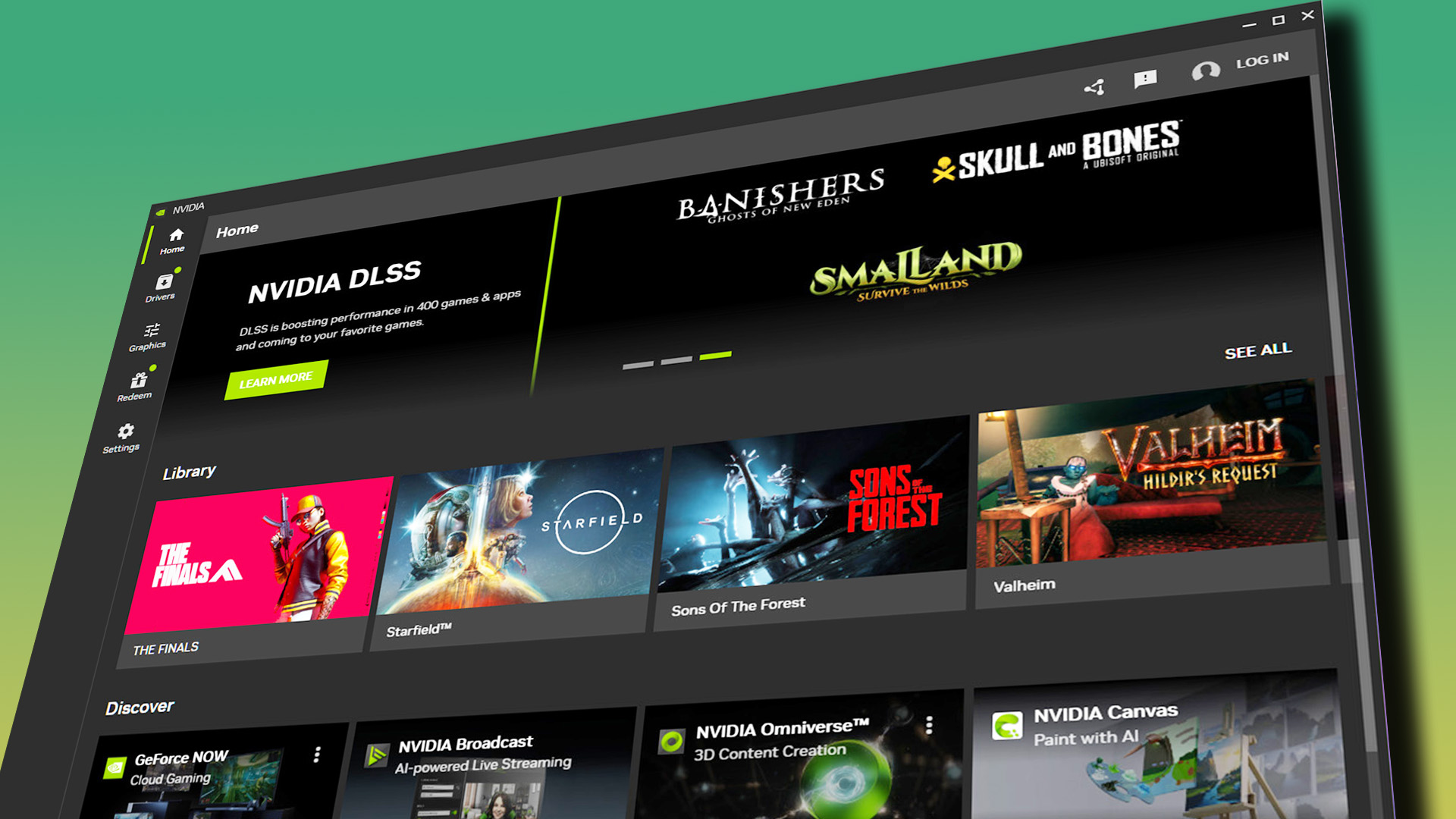This graphic appears to be a visually rich component possibly from an advertisement. The background features a blend of green and yellow-gold hues, providing a vibrant backdrop. Overlaid on this backdrop is a detailed gray website interface brimming with various elements.

At the top-left corner, prominently displayed is the word "Home" in white text. Adjacent to this is a circular icon resembling either headphones or a simplified person graphic, labeled "Log In". Further navigation icons include a white box, a white X symbol for closing, and a white minimize button.

On the side panel of the website, there is an intricate layout of icons. This includes a house icon, a small square with a play button, lines accompanied by a music note icon, a cogwheel, and several other navigational symbols.

The top of the gray website interface features another "Home" heading. Below this heading, in white font, the text "NVIDIA DLSS" stands out. A green box is present along with a multitude of graphics.

The content appears to be heavily game-oriented; titles listed in white text include "Banishers", "Skull and Bones", "Smallland", "The Finals", "Starfield", "Sons of the Forest", and "Valheim". Additionally, there are mentions of NVIDIA's services and products such as "GeForce Now", "NVIDIA Broadcast", "NVIDIA Omniverse", and "NVIDIA Canvas".

The graphic includes numerous still images with diverse themes, such as pink and blue backgrounds, faces, and a pirate ship, among other visuals.